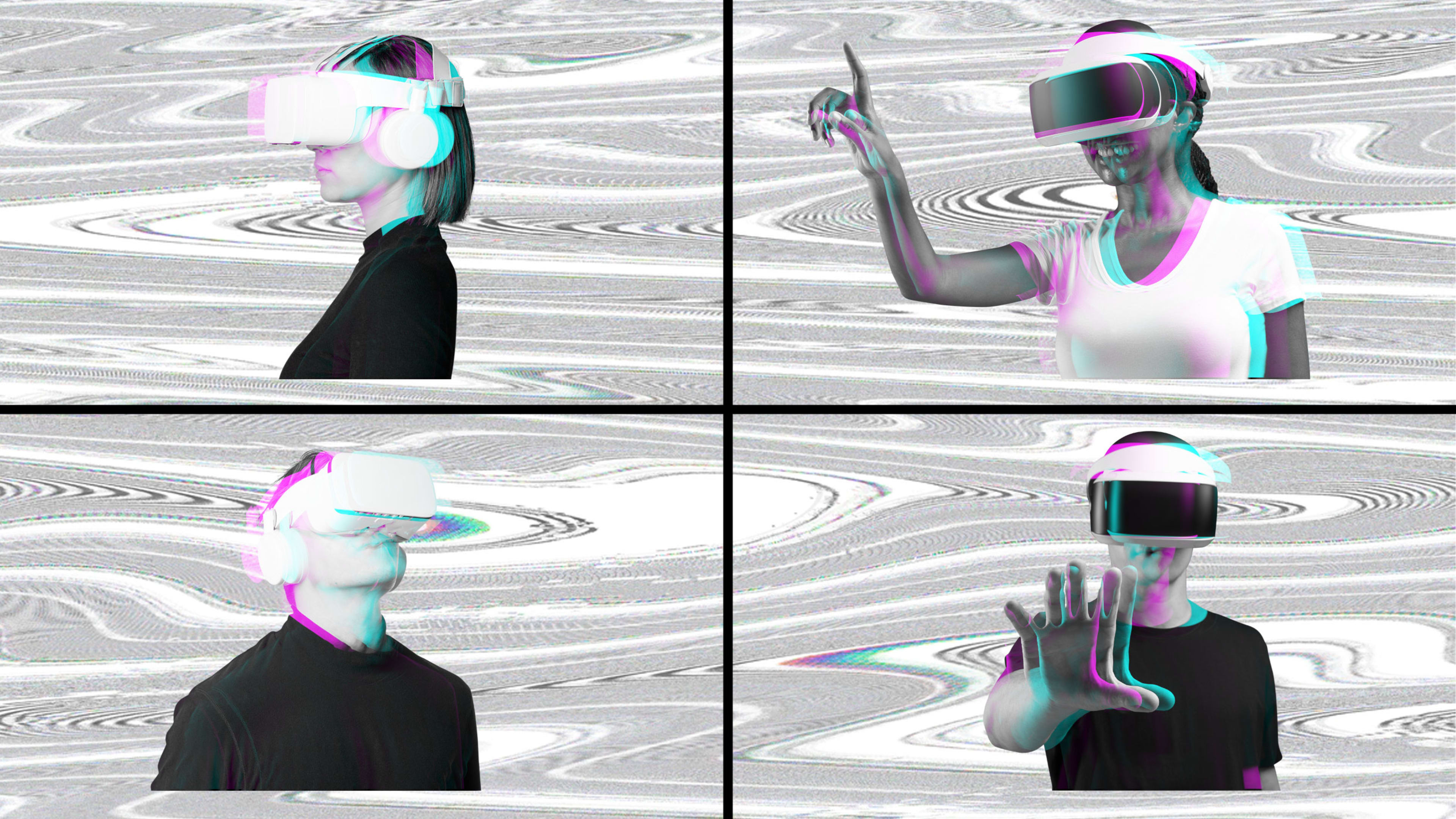The image is a 2x2 grid of four people using virtual reality headsets, each framed in a separate box against a background that resembles white distorted TV static with tinges of turquoise and magenta. In the top left frame, a white woman wearing a black shirt and a white VR headset faces to the left. To her right in the top right frame, a black woman in a white V-neck shirt also faces left, holding up her right hand and pointing upwards. The bottom left frame features a white man in a black shirt, looking to the right while wearing a similar VR headset. In the bottom right frame, a female figure, somewhat blurred, also wears a black shirt and VR headset, extending her right hand forward with fingers spread. All participants are engaged in their virtual experiences, connected by the consistent, glitchy background.